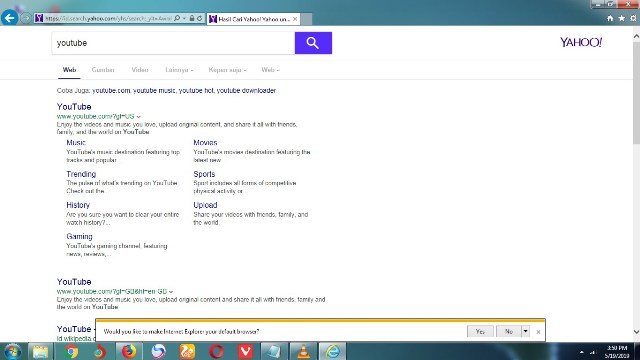This image displays a Yahoo search results page with the query "YouTube" entered in the search field. The operating system is identified as Windows 7, evidenced by the distinct taskbar icons at the bottom of the screen. These taskbar icons include File Explorer, Google Chrome, Mozilla Firefox, UC Browser, Opera Browser, Notepad, VLC media player, and Internet Explorer.